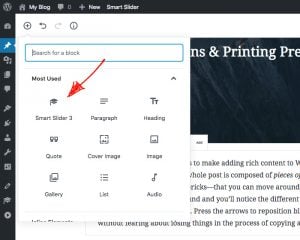A small screenshot captures the upper-left corner of a website, framed by a black border on the top and left sides. The blurred image, difficult to decipher due to its size, showcases a white background typical of the corner of a webpage. A pop-up menu with unclear text is visible, featuring a red arrow pointing to the first option on a grid of nine icons, arranged in three rows of three. Each icon has small, illegible black writing beneath it. Behind the pop-up menu, a partially visible black rectangle with white text reads "NS and printing BRE," though the full message is cut off and indiscernible. Below this, a paragraph of black text on a white background is present but not readable. Along the left side of the screenshot, several white icons are lined up on a bar, also too small to identify. At the top of this bar, a blue icon seems to be the trigger for the pop-up menu, adding to the overall navigational context of the website fragment.